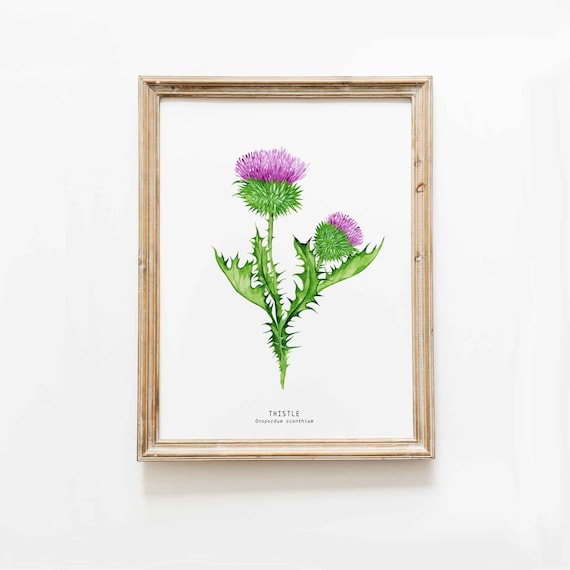The image depicts a centrally mounted painting of a thistle flower, characterized by a pink top and sharp green leaves. The painting is enclosed in a light-colored wooden frame adorned with some dark stains, enhancing its rustic look. The entire setup is placed against a solid white background which dominates the majority of the image, with noticeable shadow reflections of the frame adding depth. Notably, near the painting, there is text that reads "Sizzler, Twizzler, son," the only discernible words in the picture. The colors present in the image include beige-ish wood, green, purplish-pink, white, and black, contributing to the overall composition's clean and minimalistic aesthetic.